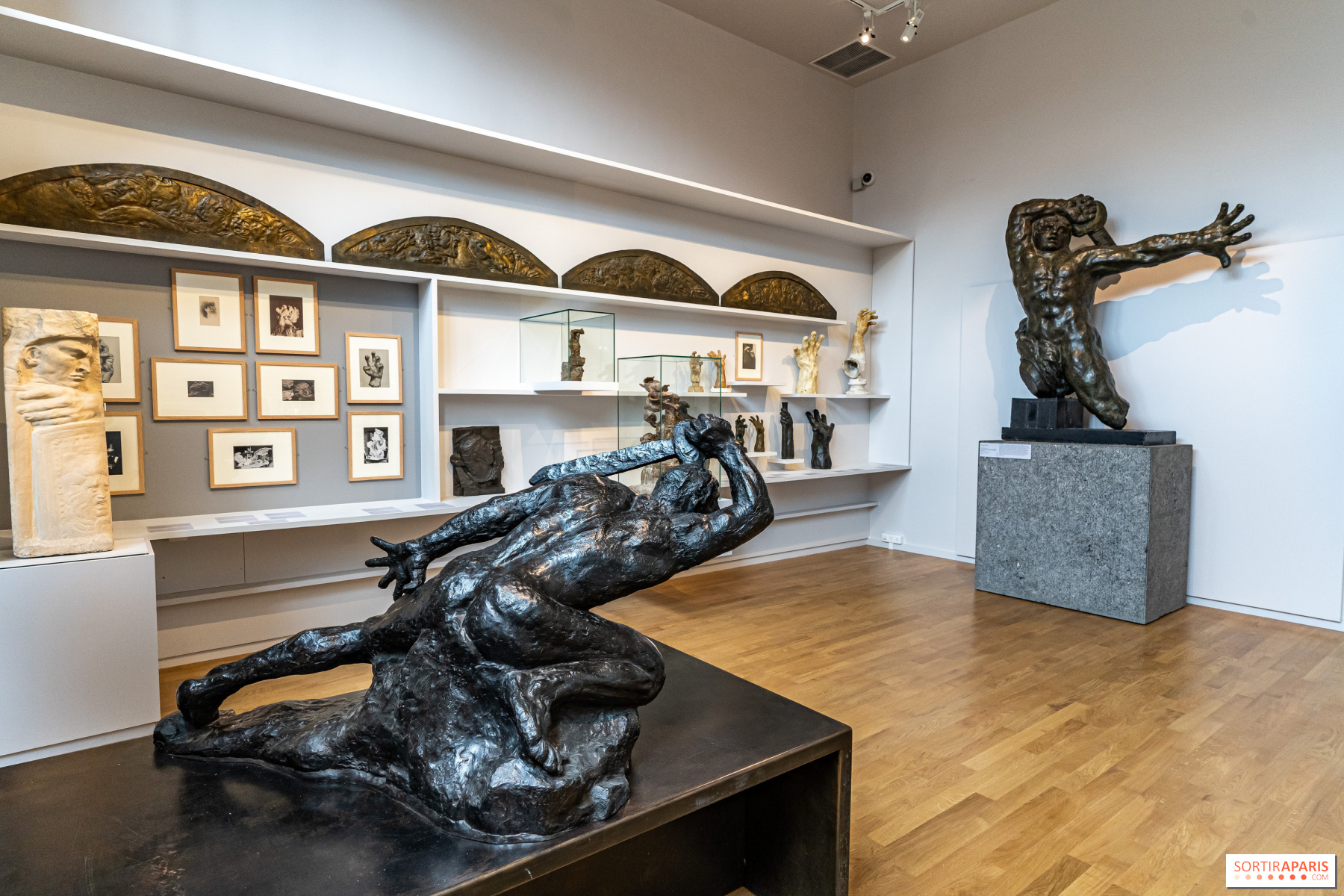The image depicts a museum gallery with hardwood floors and pristine white walls and ceilings. Dominating the room are two large sculptures of men, each holding swords and mounted on separate platforms. One prominent sculpture, positioned on a gray cement block near the wall, portrays a muscular, naked man with an outstretched arm and a sword held behind his back. His dynamic pose showcases one bent leg while the other is stretched behind him. The second sculpture, situated towards the center of the floor on a white pedestal, features a muscular, kneeling man also brandishing a sword. The gallery's walls are adorned with a variety of paintings, small sculptures, and artifacts housed on shelves and in glass cases. Notable details include gold-colored pieces, possible ancient artifacts, and intricate carvings. Overhead, spotlights illuminate the art, and an air vent is visible in the top corner, adding to the room's well-lit and ventilated atmosphere.